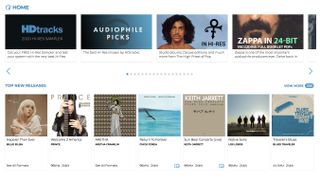The image appears to depict a small, possibly halved desktop screen with a distinct layout. At the very top of the screen is the word "Home," written in a minuscule, blue font. Below this, there are four horizontally aligned rectangular thumbnails. The first rectangle is labeled "HD Tracks," followed by "Audiophile Picks" on the second. The third thumbnail portrays a man with shoulder-length, curly brown hair next to a symbol that resembles Prince's iconic emblem. The fourth rectangle features a man's face with a mustache, his eyes cropped out, and labeled "Zappa in 24-bit."

Beneath these thumbnails is another set of text in blue, even smaller than the "Home" label, making it indecipherable. Under this text lies a horizontal row of seven square thumbnails. The first square shows a girl with blonde hair. The second thumbnail depicts a woman holding an object, possibly a guitar. The third features a pattern with a man standing at its center. The fourth square illustrates a swimming pool with a bird flying overhead. The fifth thumbnail is largely blank, save for the name "Keith something." The sixth square shows the silhouettes of five people standing outside. The final thumbnail is divided into white and blue halves with some illegible text on it.

Overall, the screen is visually divided into sections of thumbnails, each featuring various content ranging from portraits to abstract patterns.